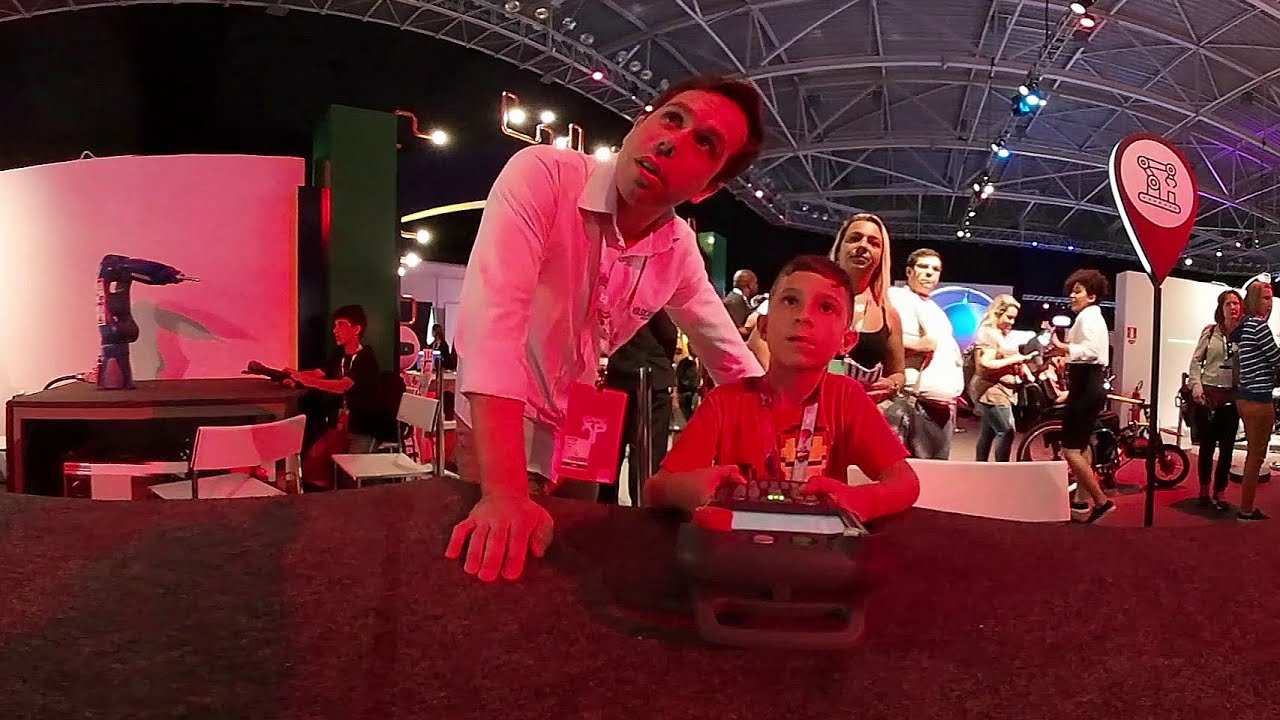In the image, a young boy with short hair and brown eyes is seated at a table, concentrating intently on a video game controller with three fluorescent green lights. He's wearing a t-shirt and his hands are positioned directly in front of him, gripping the controller. To his immediate left sits a man in a long-sleeve white shirt, adorned with a lanyard and identification card, who is also gazing slightly upwards. The man has one hand flat on the table, while his other arm extends behind the boy.

Behind them, a woman with shoulder-length blonde hair and tanned skin is wearing a black tank top and staring forward. Further in the background, another man with a large stomach, short hair, a white shirt, and black jeans is looking straight ahead while facing to the right.

The setting appears to be a convention center with a science fair atmosphere, featuring exhibits and various technological displays. One such exhibit can be seen to the far left: a large drill sitting on a wooden table, bathed in white light from the wall behind. A person is seated at the edge of the table, examining the drill while holding some papers.

The ceiling above consists of metal bars with a black backdrop, and a red, teardrop-shaped sign with a pink circle and mechanical animation is mounted on a black post to the right side of the image. The overall scene is vibrant and bustling, with multiple people in the background showing keen interest in the boy's activity, under soft red and blue lighting that enhances the lively ambiance of the event.